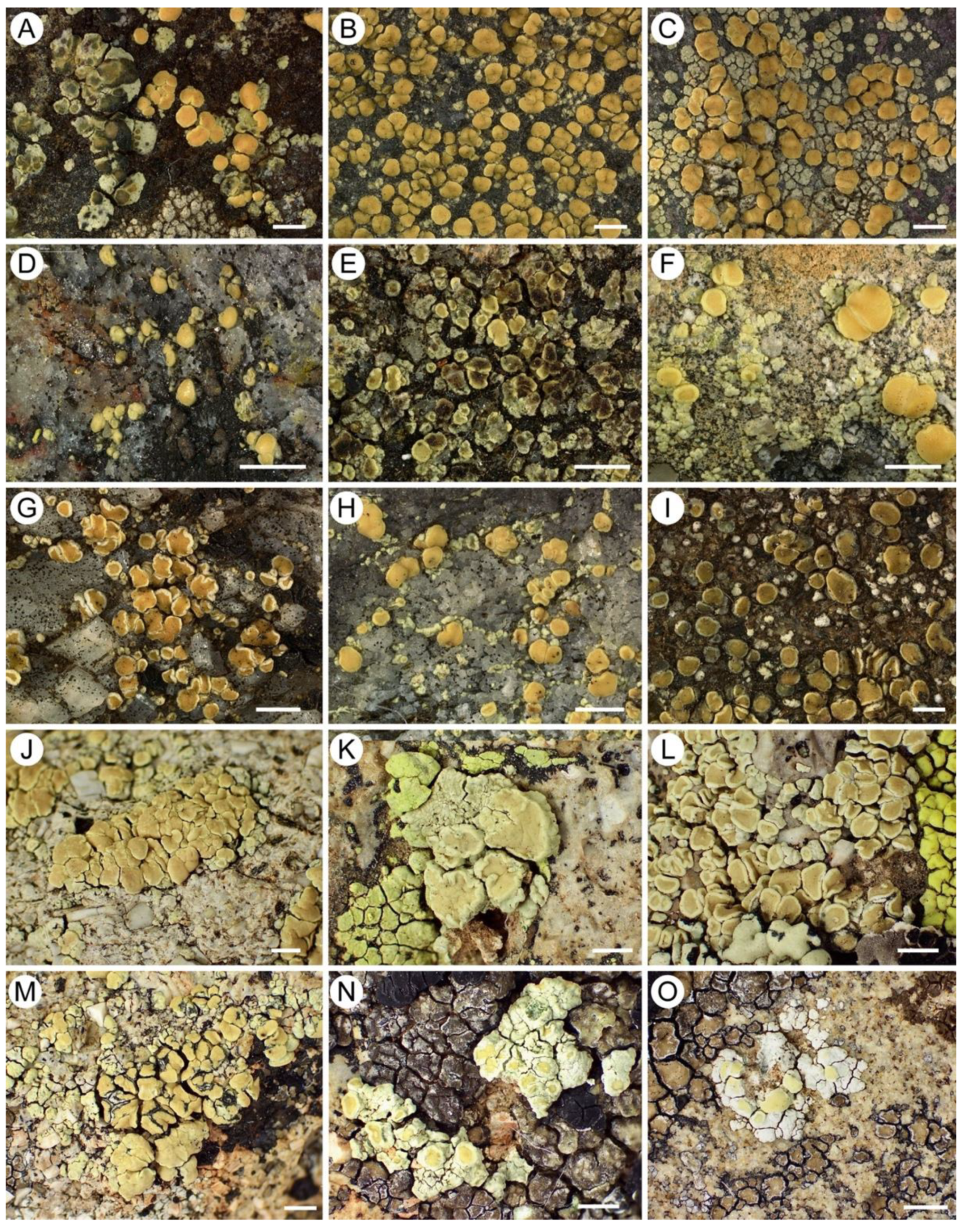The image features a photographic series of 15 side-by-side overhead shots, arranged in a 5-row by 3-column grid, depicting the growth stages of various mushrooms, lichens, or fungi on different surfaces, predominantly brown and cracked soil. Each photo is labeled from A to O, showcasing a progression from sparse to denser and more varied formations. 

- **A**: Shows the small beginnings of brown mushrooms.
- **B**: Displays an increasing number of brown mushroom tops.
- **C**: Continues with more brown mushroom tops.
- **D**: Features a few small, button-like brown mushrooms on a gray and black background.
- **E**: Illustrates some green and gray mushrooms with surrounding plants.
- **F**: Highlights larger, bulbous orange-brown mushrooms.
- **G**: Similar to F, with more bulbous mushrooms.
- **H**: Fewer, but still large brown mushrooms.
- **I**: Contains numerous dark brown mushrooms.
- **J**: Depicts an atypical fungus, without traditional cap and stalk, resembling a small brown body.
- **K**: Shows a green blob-like formation.
- **L**: Displays gray blob-like structures.
- **M**: Features yellow and brown blobs.
- **N**: Exhibits black and yellow blobs.
- **O**: Concludes with mostly yellow blobs among black and gray ones, on dryer, sparser soil.

No text other than the alphabetic labels appears in the photos, and the detailed progression captures the growth and environmental variance of these organisms.